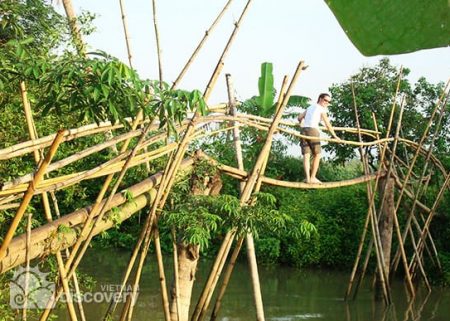In this low-quality photograph with a "Vietnam Discovery" watermark in the bottom left-hand corner, a tourist is crossing a precarious bridge made of thin bamboo poles, likely bound together to form the walkway. The bamboo handrails are tied across for support as the bridge bows slightly under the traveler's weight. The person, wearing sunglasses, a white shirt, and brown cargo shorts with their hair tied back in a ponytail, is looking back towards the camera. The bridge stretches over a murky, brownish-green body of water, surrounded by dense foliage and thick forest shrubs. A light gray sky peeks through the background, adding a serene but adventurous vibe to the image. The upper right corner of the photo is obscured by a large leaf, adding to the natural feel of the scene.